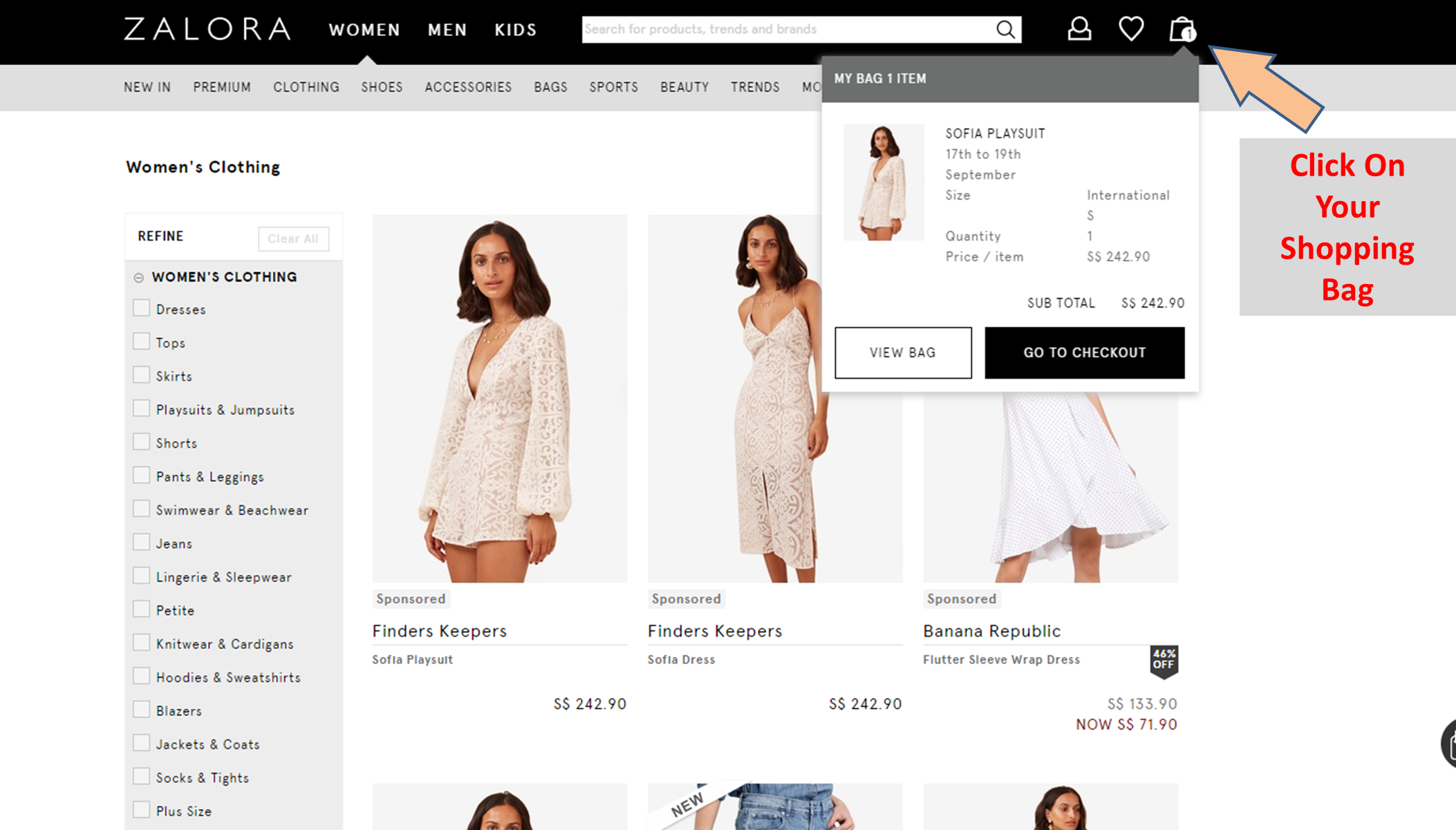The image depicts the Zalora website interface with detailed annotations. In the upper left corner of the page, the Zalora logo is prominently displayed in white font against a black navigation strip. This top strip also includes navigation links for different sections: "Women's," "Men's," and "Kids." To the right of these links lies a white search bar with placeholder text that reads, "Search for products, trends, and brands." Adjacent to the search bar's right side is a search icon.

Continuing to the right, the navigation strip features three additional icons: a person icon for user profile, a heart icon representing favorites, and an open shopping bag icon indicating one item inside. Above the bag icon, a peachy orange arrow with a blue outline points directly at it, and a gray box atop the page displays a red label with the text, "click on your shopping bag," suggesting an instructional overlay.

Upon closer inspection of the shopping bag section, it reveals details of the item inside: a "Sophia Playsuit, 7-19, September size international small quantity one," priced at $242.90, bringing the subtotal to $242.90. Below these details are two buttons: "View Bag" in a white button with black font, and "Go to Checkout" in a black button with white font. These elements are designed to guide the user through the purchase process.

Just beneath the black navigation strip, a gray bar provides additional navigational links or options. The page layout is somewhat obscured by the pop-out instructional overlay, but the described elements clearly illustrate the various functionalities available to the user on the Zalora website interface.